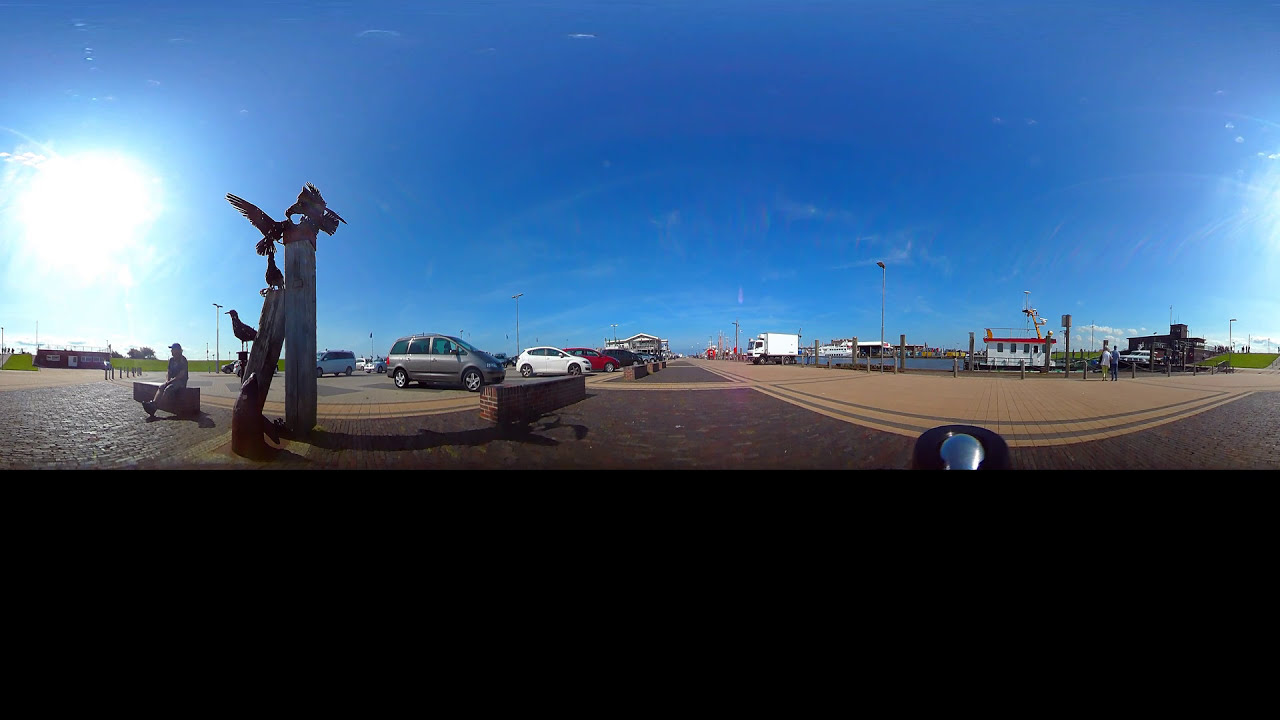The image showcases a bustling harbor-side area dominated by a large parking lot. In the foreground, a variety of vehicles including vans, sedans, small cars, and a box truck are neatly arranged. To the left, an older man in a blue shirt and hat sits pensively on a bench, gazing into the distance. Adjacent to him stands an intricate sculpture depicting birds. The scene extends to a sunny, cloudless blue sky, casting a bright light across the area.

In the middle ground, a boardwalk extends towards the ocean, partially visible with pier decking creating a nautical backdrop. A tugboat is docked to the right, equipped with what seems to be a crane, while other boats are moored further away. People can be seen walking towards these vessels, adding a lively atmosphere to the serene setting.

The parking lot itself features a pattern of dark bricks in the center bordered by lighter bricks, creating a visually appealing surface. A closer inspection reveals that there might be elements like a water spout near the left side of the image and a sun partially framed in the upper left background. The far-right background hints at a rural scene, with a possible farmhouse, a truck stop, and brown fields providing a contrasting rustic touch to the otherwise maritime environment.